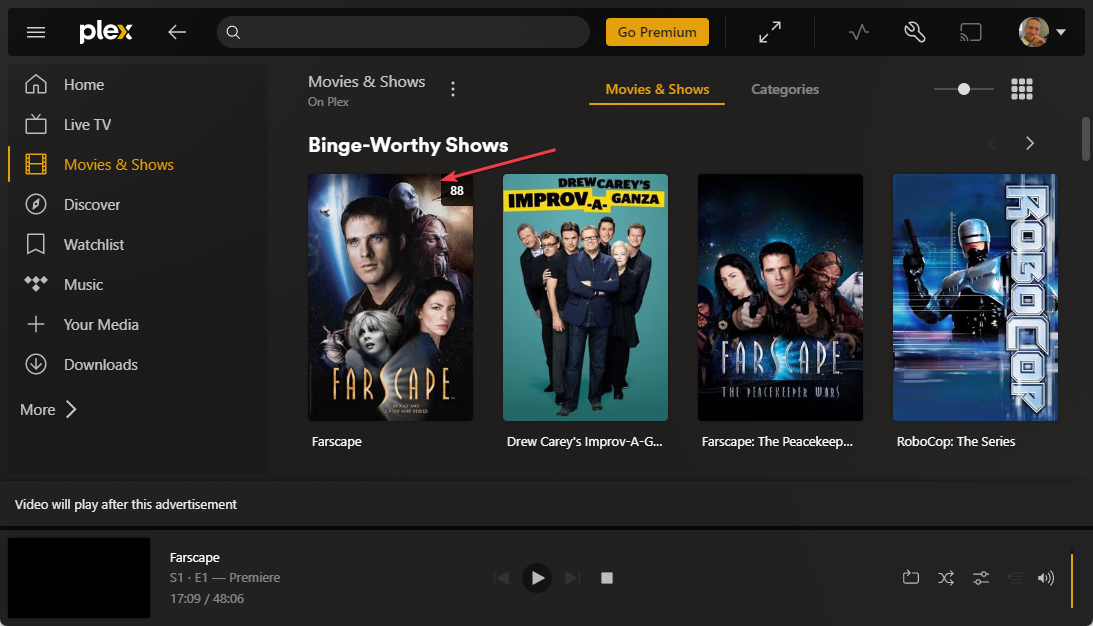In this image, we see the detailed interface of a movie streaming site, possibly its homepage. At the very top, a black rectangular border spans the width of the screen. On the left side of this border, three horizontal lines—resembling a dropdown menu—are positioned next to the Plex logo. The logo features lowercase letters, with "p-l-e" in white and the "x" split into a yellow left half and a white right half. Adjacent to the logo is a small space followed by a white, left-pointing arrow. Near this arrow is a dark gray search box with a white magnifying glass icon inside. To the right of the search box, an orange button with black text reads "Go Premium."

Continuing to the right, several icons are positioned: a full-screen icon with two outward-pointing diagonal arrows, a stock chart icon with a line that dips and then rises, a screw icon, a square icon with an audio symbol in the corner, and an avatar depicting a man's face—pale skin and brown hair—next to a downward-facing triangle.

On the left side of the image, a black navigation menu displays white text and icons. The menu items listed are: Home, Live TV, Movies and Shows (highlighted in yellow, indicating the current page), Discover, Watchlist, Music, Your Media, Downloads, and More—a right-facing caret indicates additional options.

To the right, a section with a dark gray background showcases the available shows. At the top left corner, "Movies and Shows" is written in white, with "Unplexed" below in gray. Beneath this, bold white text proclaims "Binge-worthy Shows," accompanied by show thumbnails. Featured shows include "Farscape," "Drew Carey's Improvaganza," "Farscape: The Peacekeeper Wars," and "Robocop: The Series."

At the bottom, a panel indicates video player controls within a black box. On the left, it states "Video will play after this advertisement" in white. Below, a black box placeholder represents the episode image. Information about the currently selected show, "Farscape," is provided: its title in white, "S1.E1 - Premiere" in gray, and a timestamp of "17:09 / 48:06." The control bar in the middle includes play, rewind, and fast-forward buttons, while additional options such as shuffle, settings, and volume control are located to the right.